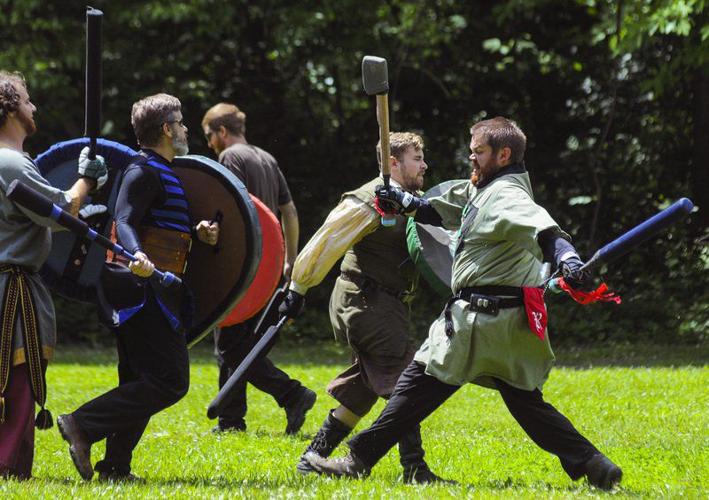In this vibrant color photograph, a group of five men are enthusiastically participating in a Live Action Role Play (LARP) session set in a grassy field on a sunny day with trees in the background. All participants are dressed in Viking-inspired garments, complete with tunics and belts. The scene depicts two men on the right, each donned in brown and white attire. The foremost man is wielding a foam axe in his right hand and a baton in his left, while the man behind him carries a green shield and a black baton. On the left side, one man is clad in a purple and black striped vest, black pants, and a black undershirt, holding a silver shield. Next to him, another man bears a purple shield and a black baton. Additionally, the man in the purple shirt also has a black and purple baton. Slightly distant from this group, there stands a fifth man holding a red shield, seemingly less engaged. The lively scene captures the essence of their immersive, playful adventure on a bright, sunny day.